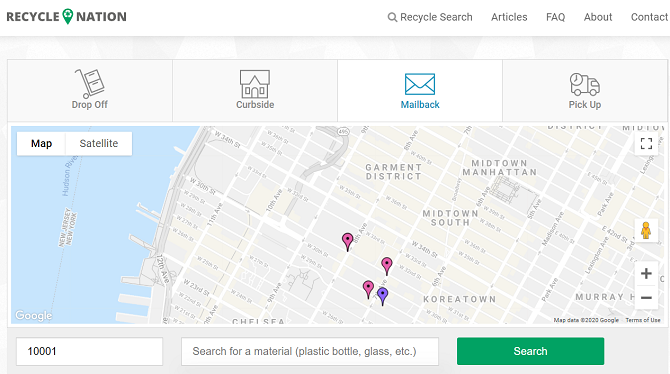Here's a detailed and cleaned-up caption for the described image:

"This is a screenshot of a website with a prominent white horizontal bar at the top. On the left corner of this bar, the word 'Recycle' is displayed in black font, followed by an ice cream cone icon and the word 'Nation.' On the right side of the bar, there is a small gray magnifying glass icon next to the text 'Recycle Search,' followed by navigation links: 'Articles,' 'FAQ,' 'About,' and 'Contact.'

Directly below the white bar is a gray bar, beneath which are four gray square icons representing different recycling options. The first icon is a wheelie bin labeled 'Drop Off,' followed by a home icon labeled 'Curbside,' an envelope icon labeled 'Mail Back' (which is selected, turning the icon blue and the background white), and lastly, a truck icon labeled 'Pick Up.'

Below this section, there is a roadmap featuring locations such as Midtown Manhattan, Garment District, Midtown South, and Koreatown, with arrows pointing to specific areas near Koreatown. At the bottom of the screenshot, another gray bar contains three search fields."